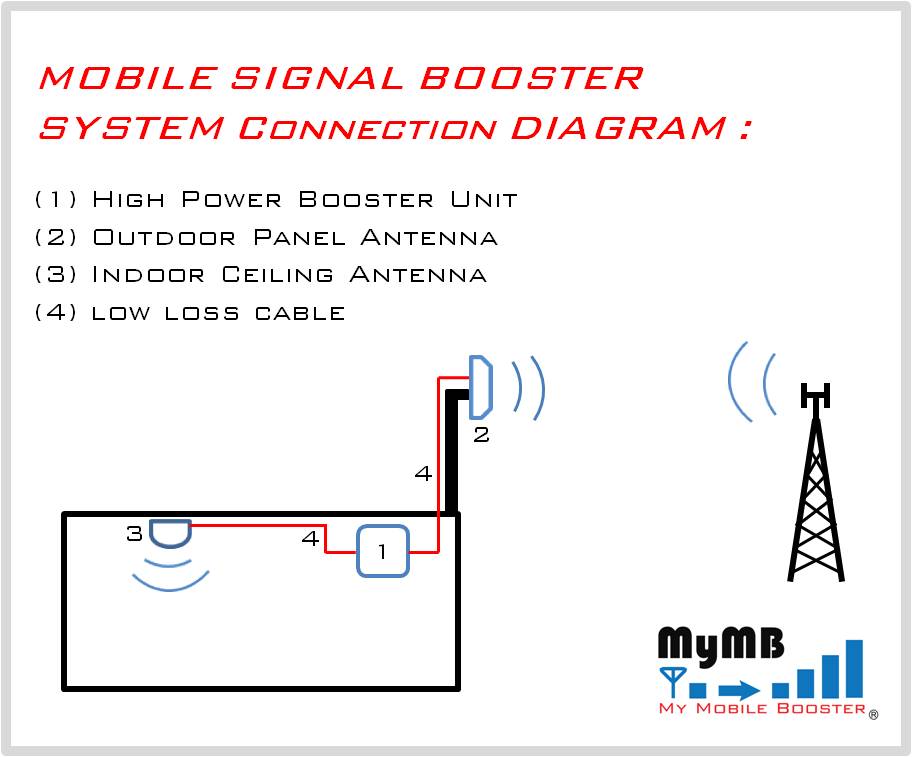The image is a rectangular informational chart titled "MOBILE SIGNAL BOOSTER SYSTEM CONNECTION DIAGRAM" in bold red text at the top. The background is mostly white, featuring multiple lines of text. Immediately below the title, a list in black text outlines four components: "1. High Powered Booster Unit, 2. Outdoor Panel Antenna, 3. Indoor Ceiling Antenna, 4. Low Loss Cable." The central portion contains a black rectangular diagram with numbered parts indicating connections: 3 (Indoor Ceiling Antenna), depicted as a half-circle with broadcasting lines; 4 (Low Loss Cable), connecting to 1 (High Powered Booster Unit), shown as a blue square; and finally extending to 2 (Outdoor Panel Antenna) on the top right sending and receiving signals to and from broadcasting lines. The bottom left corner of the diagram features a logo and watermark, "MyMB, My Mobile Signal Booster," indicating the product name.